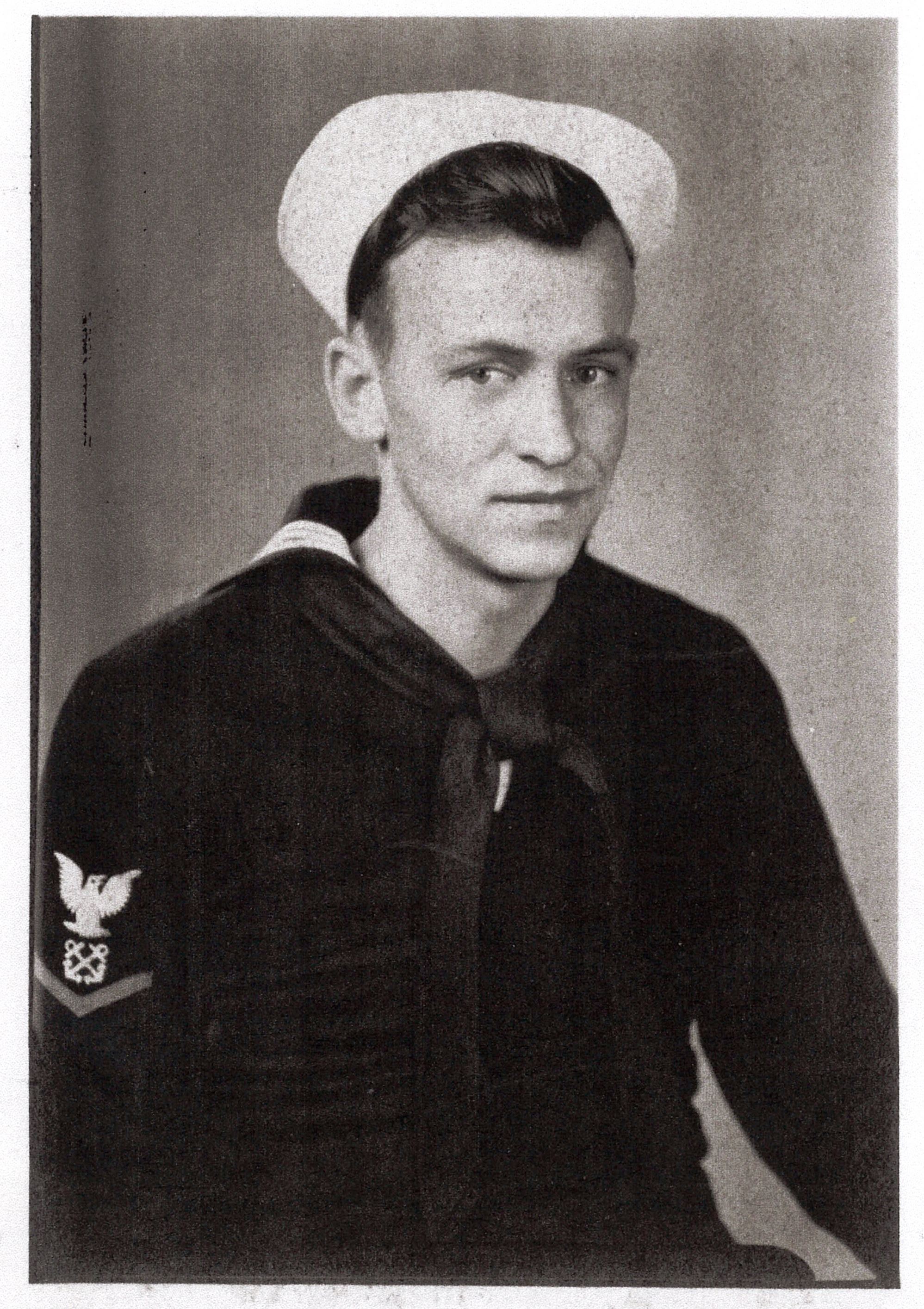This is a detailed black and white portrait from the World War II era, depicting Robert Hinsdale, a US Navy sailor from Michigan who served on the ship Pensacola and was present at Pearl Harbor. The photograph captures Robert in his Navy uniform, complete with a white sailor hat and a kerchief tied around his neck. He is seated in front of a gray wall or screen, and the pose is formal. On his left sleeve, there is an emblem featuring a white eagle with interlocking anchors and a V-shaped band beneath it, indicating his rank and affiliations.